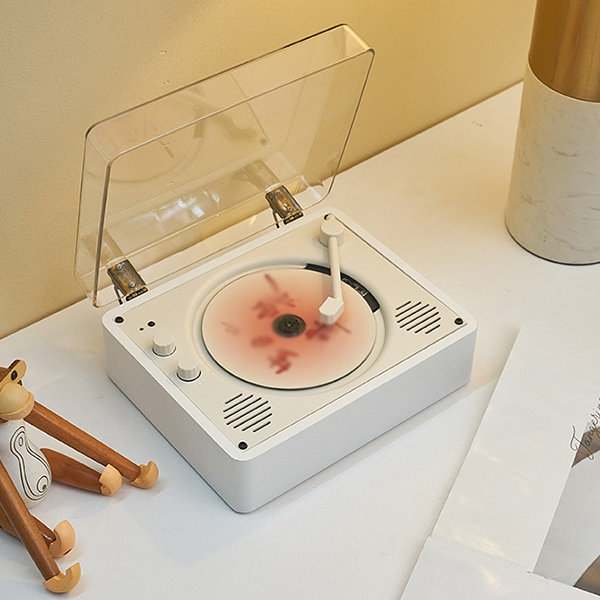The image depicts a white, portable record player with a clear hinged dust cover, sitting on a white desk against a light yellow wall. The record player, although small and possibly a toy, bears a striking resemblance to traditional models with its central platter, white tone arm, and two knobs located to the left of the platter. Intriguingly, the platter has Chinese or Japanese characters sloppily spray-painted on it. There is no vinyl record on the turntable; however, it seems a CD might be in place instead. Speaker slots are visible on either side of the player, allowing sound to emanate from it. To the left of the record player is a wooden toy monkey, and to the right is a cylindrical object featuring a white bottom and a golden top, possibly a lamp base.